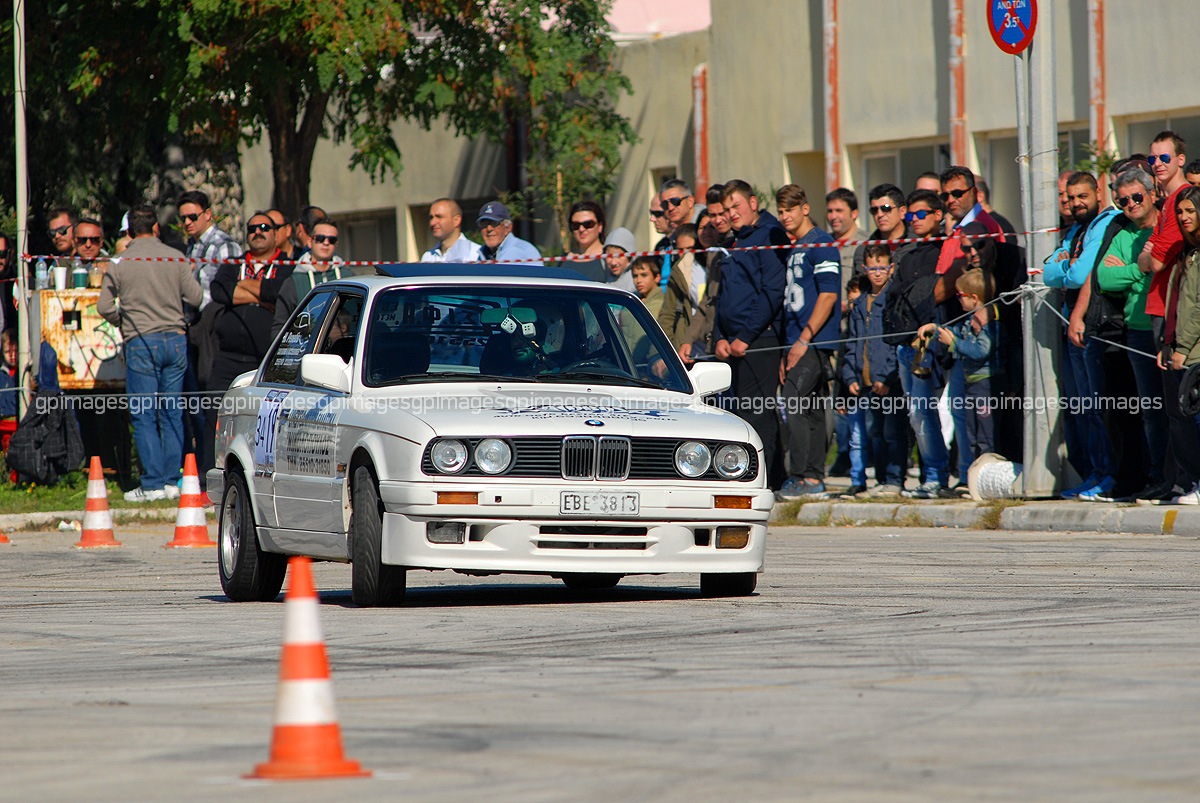A white, two-door BMW from the 1980s is maneuvering through a concrete course marked by black tire marks and three orange-and-white traffic cones, one in front of the car on the left and two behind it. The car, which is adorned with various graphics on the hood, passenger-side door, rear passenger window, and rear windshield, features four circular headlights, a black grille, a white bumper, and a white faded license plate reading EBE3813. Silver rims glint from the tires, and a pair of dice hang from the rearview mirror. As the car tilts slightly to the right while moving forward, it navigates around the cones, suggesting a possible drift or racing event. 

In the background, a diverse group of spectators—ranging from children to older adults—stand behind makeshift fencing made of red, white, and silver strings, tethered between two poles to keep them off the course. Many people have their hands resting on the string barrier. Among the crowd, a person appears to be selling drinks. Behind the crowd is a light gray building with fading white paint on its columns and sections of orange, possibly a large office or factory building. A large tree with green and some brown leaves looms in the upper left corner. On a pole to the right side of the image, a circular sign with a red outer ring, a blue center with a red "X," and "3S" in white letters is visible, indicating parking or traffic regulations. The atmosphere suggests a warm, summer day given the short sleeves worn by many in the audience.